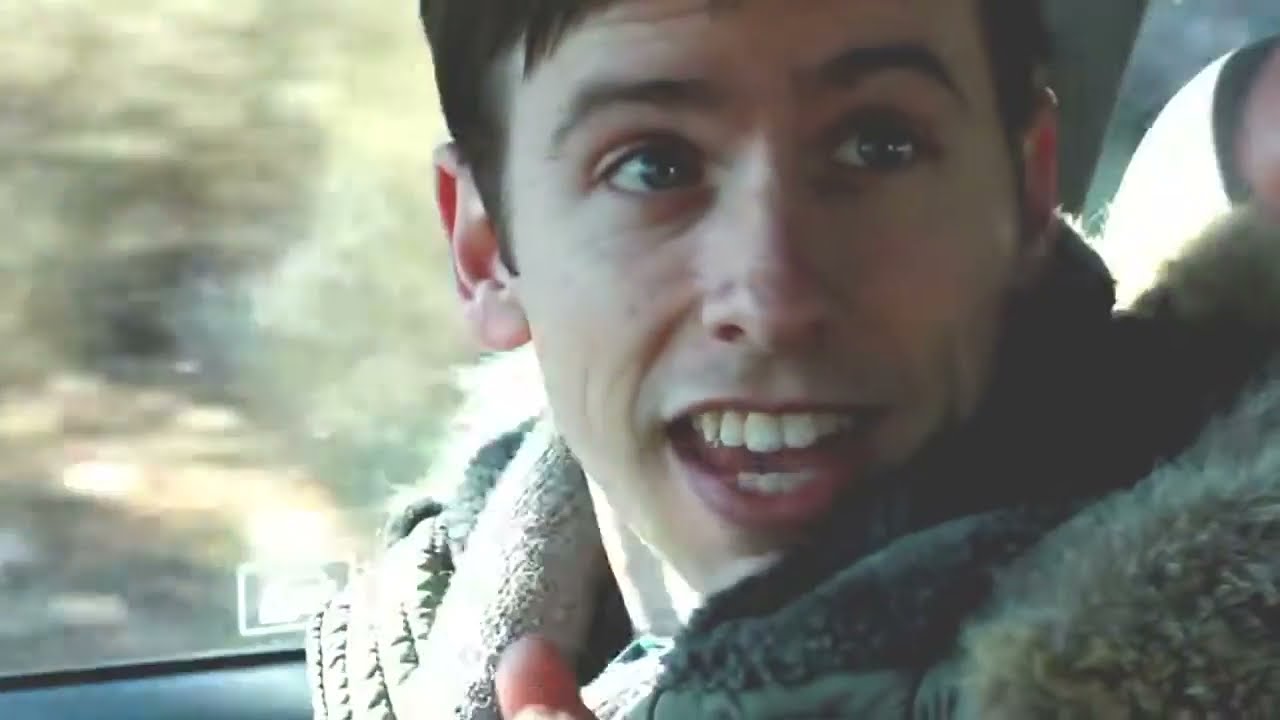This image is a photorealistic close-up of a young man with white skin, dark eyes, and short brown hair, sitting in a vehicle. His face, positioned slightly to the right of the center, is animated with his mouth open as if in mid-speech, and he appears to be looking toward the right side of the frame. The man's expression suggests excitement or engagement in a conversation, with visible movement from the top parts of his fingers indicating he might be talking with his hands. He is wearing a jacket with a fur-lined hood which is primarily gray, creating a textured contrast against the softer background. Behind him, the blurred background seen through the car's window displays indistinct but colorful hints of trees and foliage, suggesting motion. This composition emphasizes the lively and dynamic expression of the man within the confines of a moving car.